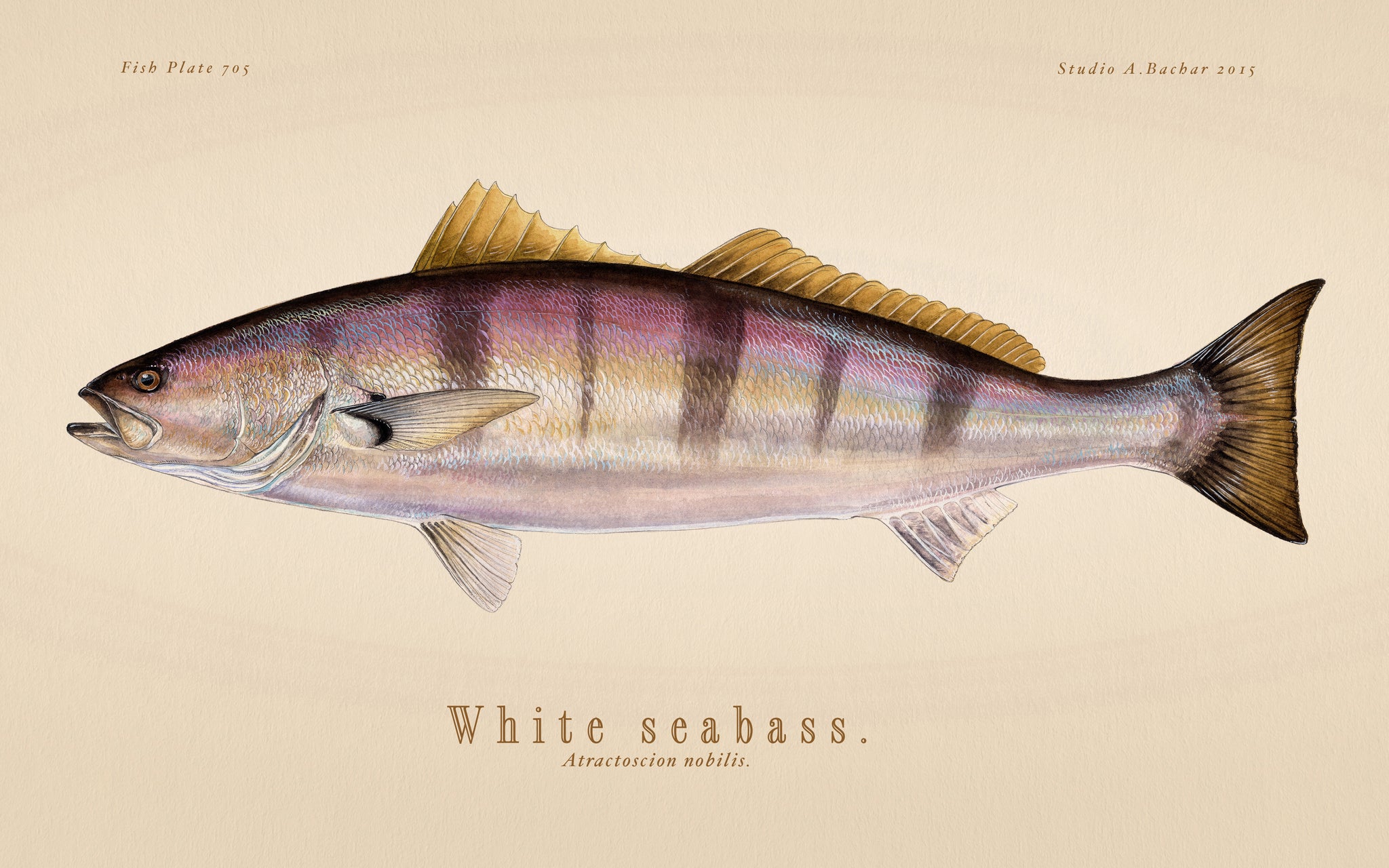The image features a meticulously detailed, hand-drawn illustration of a white sea bass, positioned centrally against a tan background. The fish's head points to the left while its tail extends to the right. Vibrant hues of purple, pink, blue, white, and gold adorn its scales, accompanied by distinctive black and brown stripes running from its back to its belly, resembling a glutinous texture. The fins exhibit a mix of yellow on the top and white on the bottom. The fish has its mouth open, showcasing a realistic yet artistic depiction.

At the top left corner, the text "Fish Plate 705" appears in a brown font. The top right corner displays "Studio A Bacaw Bacher 2015" in the same brown font. Below the fish, the phrases "White Sea Bass" and its scientific name "Atractosianobilis" are inscribed in a more formal brown font. This comprehensive rendering captures both the realistic intricacies and artistic nuances of the fish.